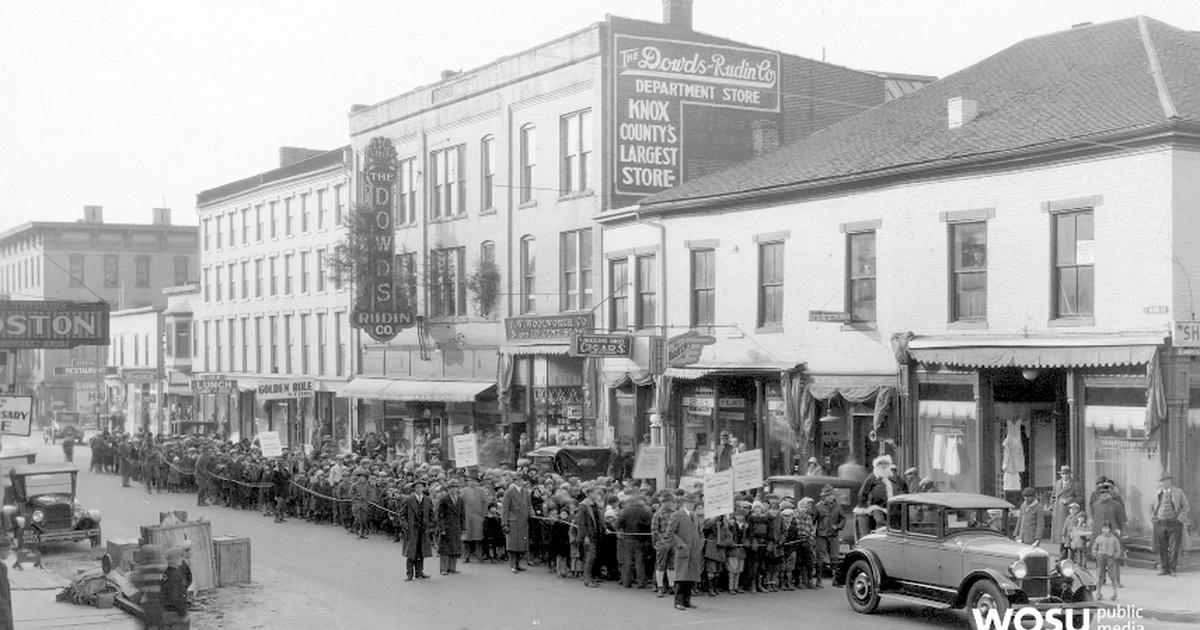This black-and-white image, likely from the 1920s or 1930s, depicts a bustling downtown street scene. In the middle section of the image, from the left to the right, we see a large number of people lined up, creating a significant crowd outside the Dowd's Rodin Company Department Store, which is prominently labeled "Knox County's Largest Store." The crowd is contained behind a barrier made of chains or ropes, suggesting an event or promotion. Many individuals are dressed in period-appropriate coats and hats, adding to the historical ambiance. Among the vintage cars parked along the street, one notable vehicle, possibly a truck or car, features Santa Claus on its back. While some individuals hold up signs, others seem to be directing the crowd. The storefront to the right displays clothing either in the window or hanging outside, contributing to the lively and organized scene. Toward the bottom of the image, the words "WOSU Public Media" are visible, likely identifying the source of the photograph.